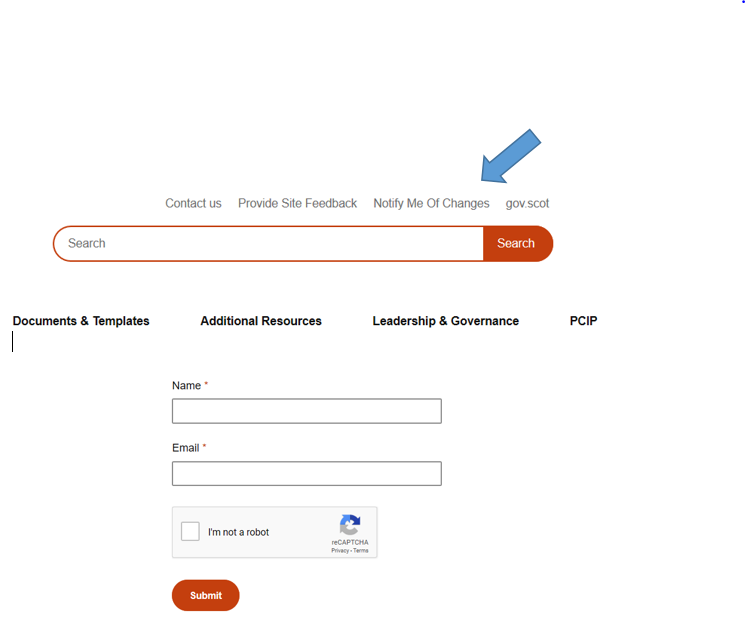This image is a screenshot taken from a computer or phone displaying a web page, specifically a search or contact page. At the top of the screen, there are several links in small print: "Contact Us" on the left, "Provide Site Feedback" to the right of it, followed by "Notify Me of Changes". A digitally-added blue arrow points downward to the "Notify Me of Changes" link in the upper right area.

Just beneath this section, there is a search bar. The search bar has a distinctive design, with a red outline and the word "Search" in gray letters on the left. The right part of the search bar has a red background with the word "Search" prominently displayed in white letters.

Further down the page, there are several headings and sections in black print. These include "Documents and Templates" on the next line, followed by "Additional Resources", "Leadership and Governance", and "Governance". Below these headings, the text continues with "PCIP". Directly under this, there are labeled input boxes for "Name" and "Email". 

Finally, there is a reCAPTCHA section with the statement "I'm not a robot", accompanied by a checkbox, and a submit button which stands out in red at the bottom of the form.